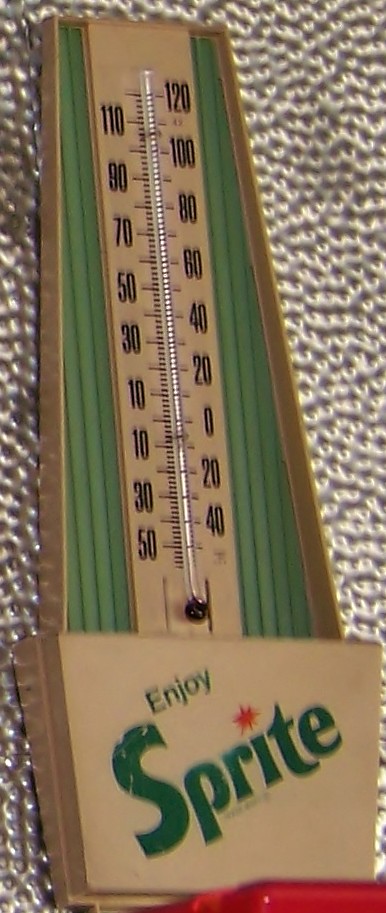This image features a vintage Sprite mercury thermometer, likely from an earlier era. The thermometer is affixed to a metal surface that has a heavily textured appearance, resembling wear from being struck by BB pellets. The metal surface, though indented and weathered, provides a rustic background for this nostalgic piece. The thermometer itself bears the cheerful slogan "Enjoy Sprite" at the bottom, hinting at its former pristine white paint, now faded to a yellowed or off-white hue due to age. Although the specific temperature reading is obscured, the thermometer's range is impressively broad, spanning from 120 degrees Fahrenheit down to 50 degrees below zero, with faint notches indicating it may even measure temperatures as low as 60 below. The mercury within the thermometer appears intact, a testament to its durability over the years.